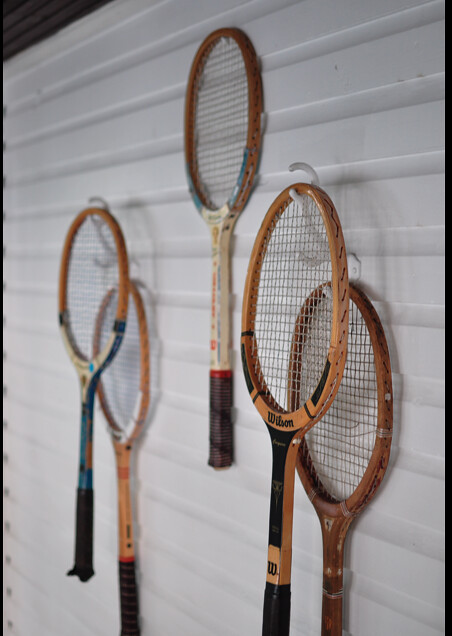This photograph depicts a collection of five old wooden tennis rackets neatly hung on a white, horizontally ridged wall, possibly resembling the interior of a garage. The rackets are suspended from sturdy white metal hooks, with some hooks appearing to be double hooks. The most prominent racket in the front proudly displays the Wilson brand, identifiable by its black markings and distinct 'W' logo. This Wilson racket is in relatively good condition, featuring a yellowish-brown wooden frame and a black rubber grip. The rackets, arranged almost in an Olympic ring pattern, exhibit a variety of color accents: blue, red, white, and black. The racket located centrally showcases blue and white markings with some blurry text, while others are characterized by walnut or reddish-brown hues and similarly dark grips. Above the display, in the upper left corner, a small triangular segment of a darker, ridged roof can be seen, contrasting against the clean lines of the white wall. The detailed arrangement and diverse coloration of the rackets highlight their vintage charm and unique craftsmanship.